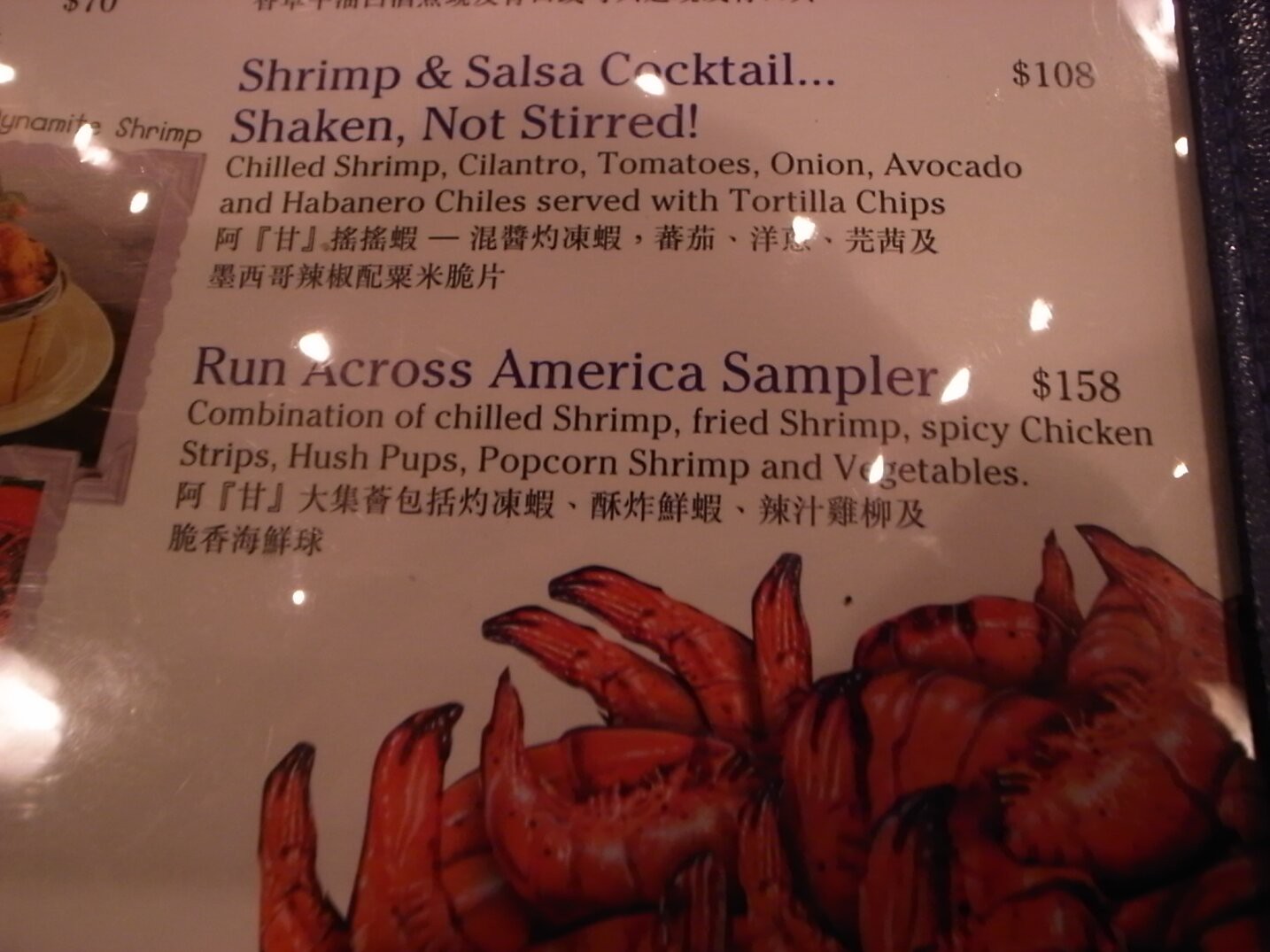This photograph captures a section of a restaurant menu encased in plastic, likely part of a leather-bound booklet commonly used to hold multiple pages of menus. The visible page features two distinct food offerings accompanied by text descriptions and prices. 

The first item listed is a "Shrimp & Salsa Cocktail—shaken, not stirred! It includes chilled shrimp, cilantro, tomatoes, onions, avocado, and habanero chiles, served with tortilla chips. Below this description, characters in what appears to be an Asian language, likely Chinese, provide a translation. The price for this dish is $108.

The second offering is the "Run Across America Sampler," a combination platter featuring chilled shrimp, fried shrimp, spicy chicken strips, hushpuppies, popcorn shrimp, and vegetables. This description also has a corresponding translation in a foreign language beneath it. The price for the sampler is $158.

In the foreground, close to the camera, there is a printed photograph of cooked shrimp, adding a visual appeal to the menu. The left edge of the menu page features a partial image of another dish, possibly "Dynamite Shrimp," as suggested by the visible text "enamite shrimp." This section shows the edge of a plate with an orange-colored item, likely part of the dish in question. 

Overall, the menu presentation combines detailed food descriptions, multilingual translations, and vibrant images to entice diners.